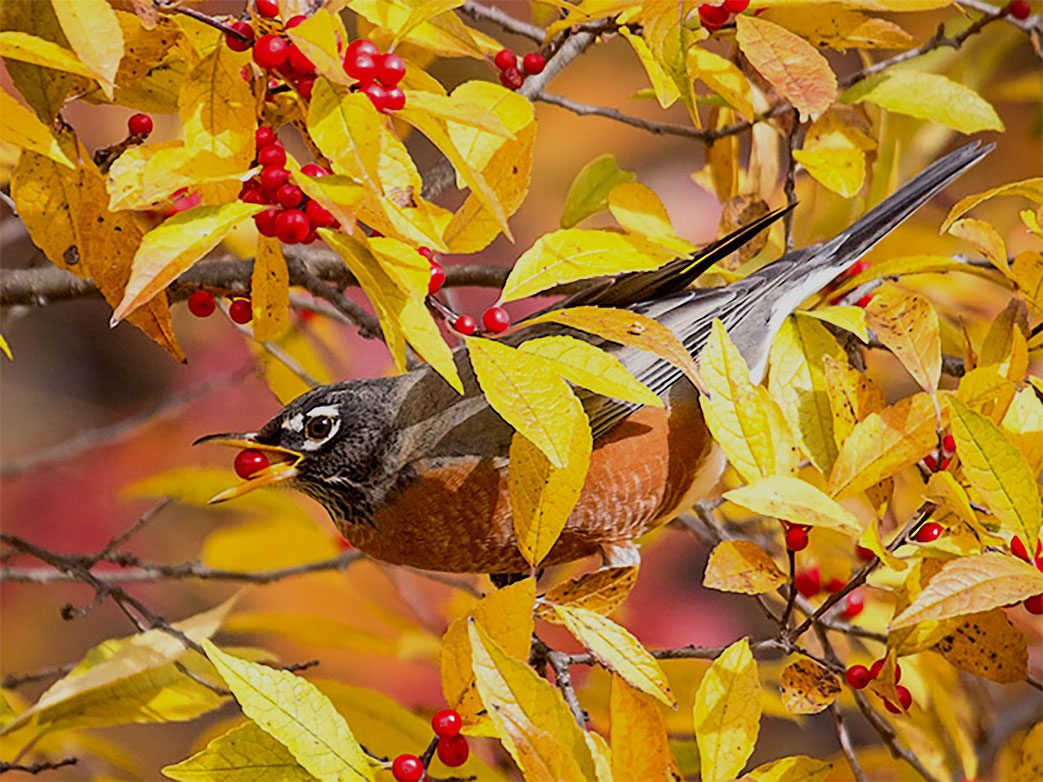A small sparrow-like bird is perched on a slender tree branch amidst a backdrop of rich autumn colors. The tree's yellow leaves, tinged with brown, signal the fall season. The bird's red crest stands out against its coat of black, gray, and brown feathers, with a splash of white around its eyes and tail. Its keen brown eyes focus on the juicy red berry clasped in its yellow and black-tipped beak. The bird appears mid-snack, attempting to swallow the bright berry. The background is notably out of focus, employing a bokeh effect that adds a blurred, dreamy quality to the scene. This depth contrasts sharply with the detailed portrayal of the bird and branches, possibly suggesting the use of digital tools in the rendering of this image, lending it a painting-like quality.